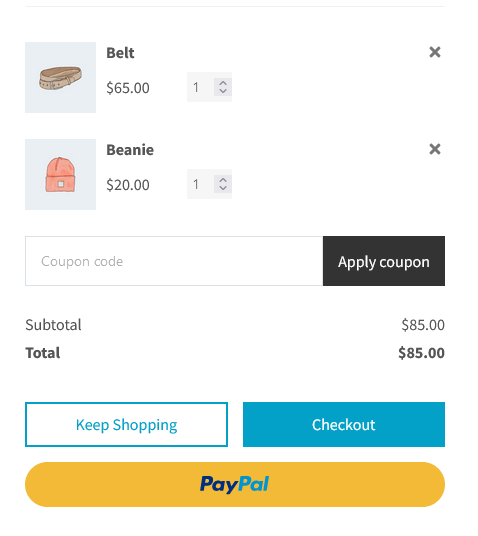The online shopping cart displays two items with detailed descriptions and pricing. 

On the left, a gray square background highlights a beige belt with a rustic tan finish. To the right of the image, "Belt" is written in bold black lettering, followed by a price of $65 in standard gray text. Adjacent to this, a gray box features a number "1" flanked by up and down arrows indicating adjustable quantity, next to a gray "X" symbol for item removal.

Below the belt, a light gray box presents a peach-colored beanie with a central gray square containing white text. "Beanie" is labeled in bold black letters with a price of $20 in gray text beneath. Like the belt, an adjacent quantity selector with up and down arrows shows "1," alongside a gray "X" for removal.

Underneath the items, a section for coupon code entry is outlined in light gray, with light gray text inside the box. To the right, a black rectangle with white text prompts users to "Apply Coupon."

At the bottom, the subtotal is listed as $85, leading to a bold "Total" of $85. Additionally, the lower left features a white rectangular icon outlined in blue with the phrase "Keep Shopping" in blue text, inviting users to continue browsing.